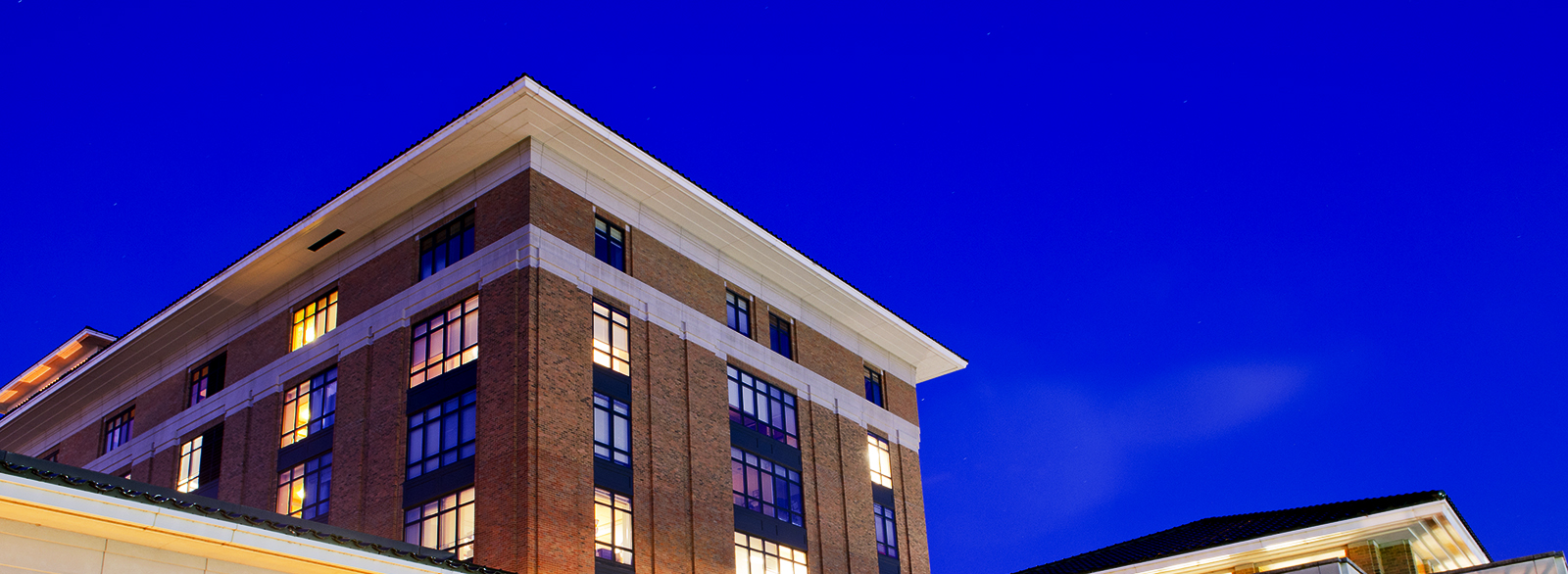This photograph captures the upper segment of a tall building, likely an office or hotel, framed within a long, rectangular image oriented horizontally. The vibrant, deep blue sky serves as a striking backdrop to the building which appears to be at least eight or nine stories tall, although only the top four floors are visible. The structure is characterized by its brown brickwork and numerous windows, some illuminated in shades of blue, red, and purplish hues, suggesting varied lighting conditions inside. The roof is flat and white, possibly constructed from wood. The image is devoid of identifying text or people, emphasizing the building's distinct, almost arrowhead-like form against the bright sky.